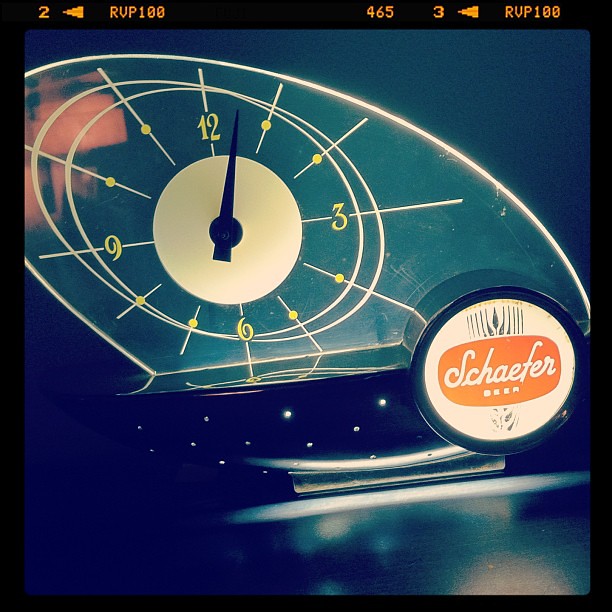This image is a detailed screenshot featuring an analog clock positioned towards the upper left corner. The clock, likely a photograph of a real clock, stands out against a bluish background. The lower portion of the background transitions into a darker blue, embellished with a few scattered stars. The clock itself has a clear surface, possibly made of plastic or lucite, with white circular markings around the face. The clock's center is a light cream color, and it features standard numbers, limited to 12, 3, 6, and 9, with lines marking the other hours. The time shown is approximately 12:03. In the lower right-hand corner, the brand name "Schaeffer Beer" is clearly visible.